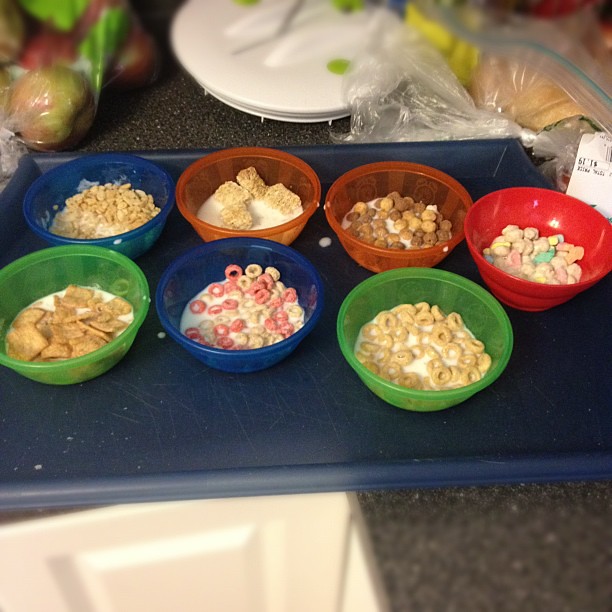In this detailed photograph, there is a slightly transparent blue tray centrally placed on a black tabletop, showcasing seven bowls of cereal arranged in two rows. The first row, from left to right, features a partially translucent dark blue bowl filled with rice flakes, a slightly transparent orange bowl with wheat cereal, another orange bowl containing Reese's Puffs, and a solid red bowl holding Lucky Charms. The second row starts with a slightly transparent green bowl filled with a different kind of cereal, a slightly transparent blue bowl that appears to contain strawberry Oreos, and ends with another translucent green bowl filled with regular Cheerios.

The blue tray rests on a black table that has some white spots. Surrounding the tray, the scene includes some additional elements: to the top left of the image, there is a bag of apples, while to the top right, there are some slightly blurry groceries including a Ziploc bag and a price marker indicating $1.29. White cabinets are visible below the tabletop, suggesting the setting is likely a kitchen. The photograph has a mix of sharp and slightly out-of-focus areas, with the foreground cereals and bowls being the most prominent elements.